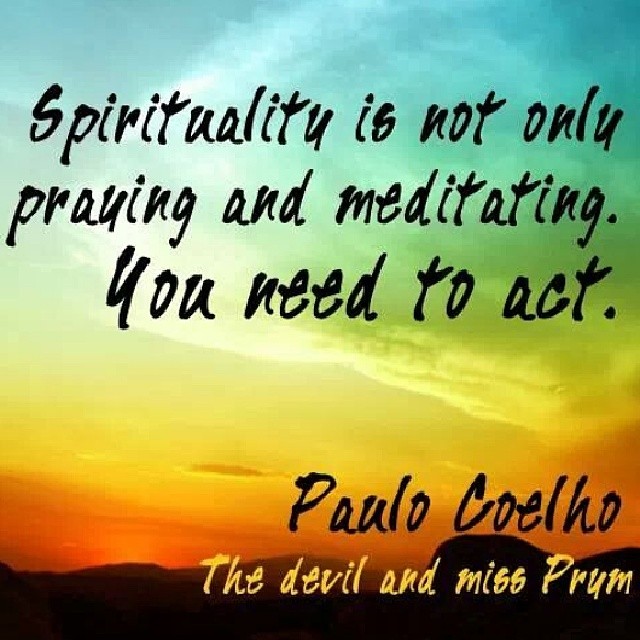The image is a square-format photograph enhanced with graphic design and typography, featuring an inspirational message. The background showcases a serene sunset landscape with blue and green sky hues fading into yellow, orange, and dark orange, accompanied by light white clouds. Silhouettes of hills, rocks, and dirt dominate the foreground, adding depth to the scene. At the top of the image, in a handwritten black font, is the motivational text: "Spirituality is not only praying and meditating. You need to act." In the bottom-right corner, the author's name, Paolo Coelho, is displayed in black letters, with the title "The Devil and Miss Prym" in a cream-colored font beneath it. The picture blends elements of realism, representationalism, and graphic design to convey its message.